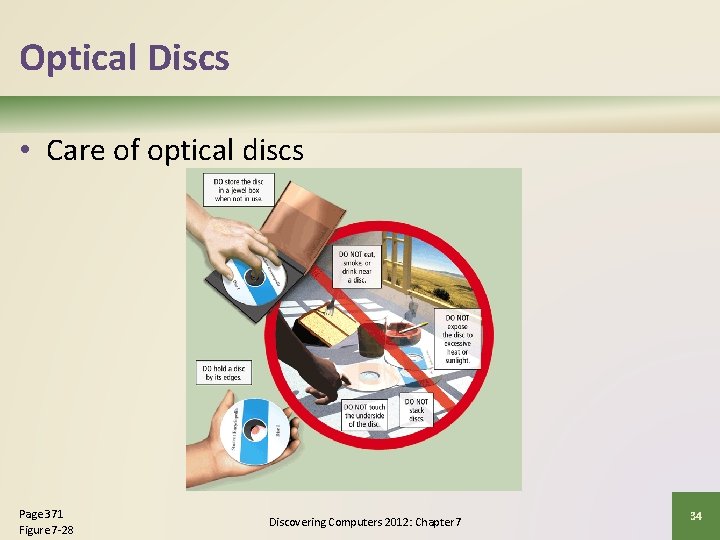The image appears to be a slide or page from a textbook or presentation on "Discovering Computers, 2012, Chapter 7." It features a white cream background with a large, light purple heading that reads "Optical Disks" in the upper left corner. Below this heading, a green bold line serves as a border, under which there is a black bullet point stating "Care of Optical Disks." 

Central to the slide is a green box containing images and text outlining proper handling of CDs. The top image within the green box depicts a hand placing a blue and white striped CD into an open CD case, with small, unreadable text beside it. Further down, there is an illustration featuring a red prohibitive circle with a line through it, overlaying images of CDs on the ground, a brush, a hand touching one of the CDs, a glass with a dark liquid, and a cigarette in an ashtray with sunlight streaming through an open window. This signifies actions that should not be taken with CDs, reinforced by partial readable text within the circle saying "do not."

The slide is detailed with references: the bottom left corner notes "page 371, figure 7-28," while the bottom center reads "Discovering Computers, 2012 Chapter 7." Finally, the bottom right corner houses a green box labeled with the number "34," indicating either a page or section number.